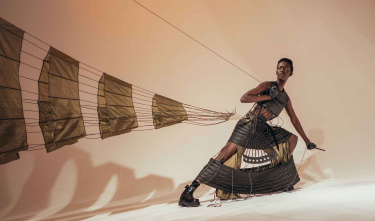The artwork depicts a black individual, commonly perceived as a man by one viewer and a woman by others, who is leaning forward at a sharp angle. This person, with short dark hair, is standing on a white surface against a pink or light orange background. They hold a piece of rope extending from their left arm, which attaches to a much longer rope connected to a fabric kite that streams back and to the left. The kite is constructed from a brown, possibly ripstop fabric, and resembles a cone or parachute-like shape. The figure's outfit is an ancient or unusual garment in shades of gray and brown, incorporating a quilted black leather appearance with interconnected pieces by wires or cables. This distinctive attire includes a sleeveless cropped top, a skirt above the knees, and leg coverings around the shins or ankles, completed with black leather combat boots. The scene is artfully lit, casting shadows onto the background, and the figure leans into the tension of the kite with a dynamic and forward-reaching stance.